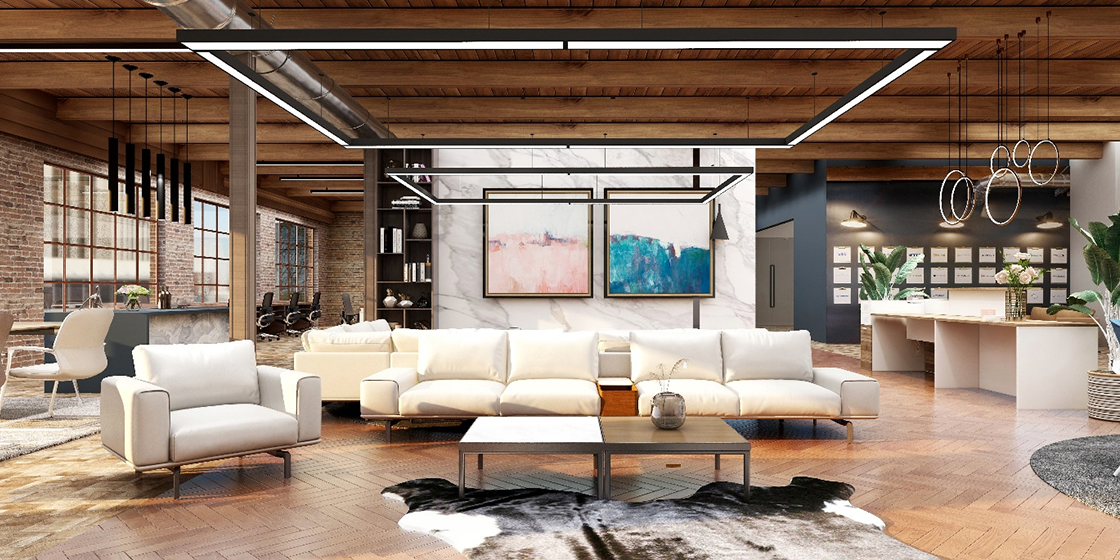The image captures a meticulously designed, modern, warehouse-style living space with an industrial flair, reminiscent of a repurposed commercial property typical in downtown New York. The room features an open-plan layout with natural brick walls on the left and a combination of navy blue and gray painted walls on the right. The ceiling showcases exposed wooden beams with recessed wooden panels, adorned by large square lighting fixtures and a unique circular light fixture.

In the foreground, a large white sectional couch with smaller black-legged seats is centrally positioned, complemented by a matching armchair on the left. Two butted coffee tables—one white, the other with a brown surface—sit atop a black fur-patterned rug. The spacious room also includes a wooden-patterned zigzag floor, adding to the overall rustic yet modern aesthetic.

Toward the back, there is a white granite wall serving as an island divider, featuring two abstract paintings—one with a pink and white scheme, the other in blue and white. Adjacent to this wall is a bookshelf filled with books and knick-knacks. The far-left corner reveals a bar or kitchen counter area framed by large grid windows, while the right side of the room houses a long white desk with a wooden top, set against a navy blue wall adorned with numerous printed items and topped by ring-shaped lights.

Additional elements include various plants and flowers strategically placed around the room, enhancing the natural ambiance. The overall scene is highly staged, exuding a catalog-like perfection with minimal personal effects, suggesting a stylish, multi-functional living or office space.